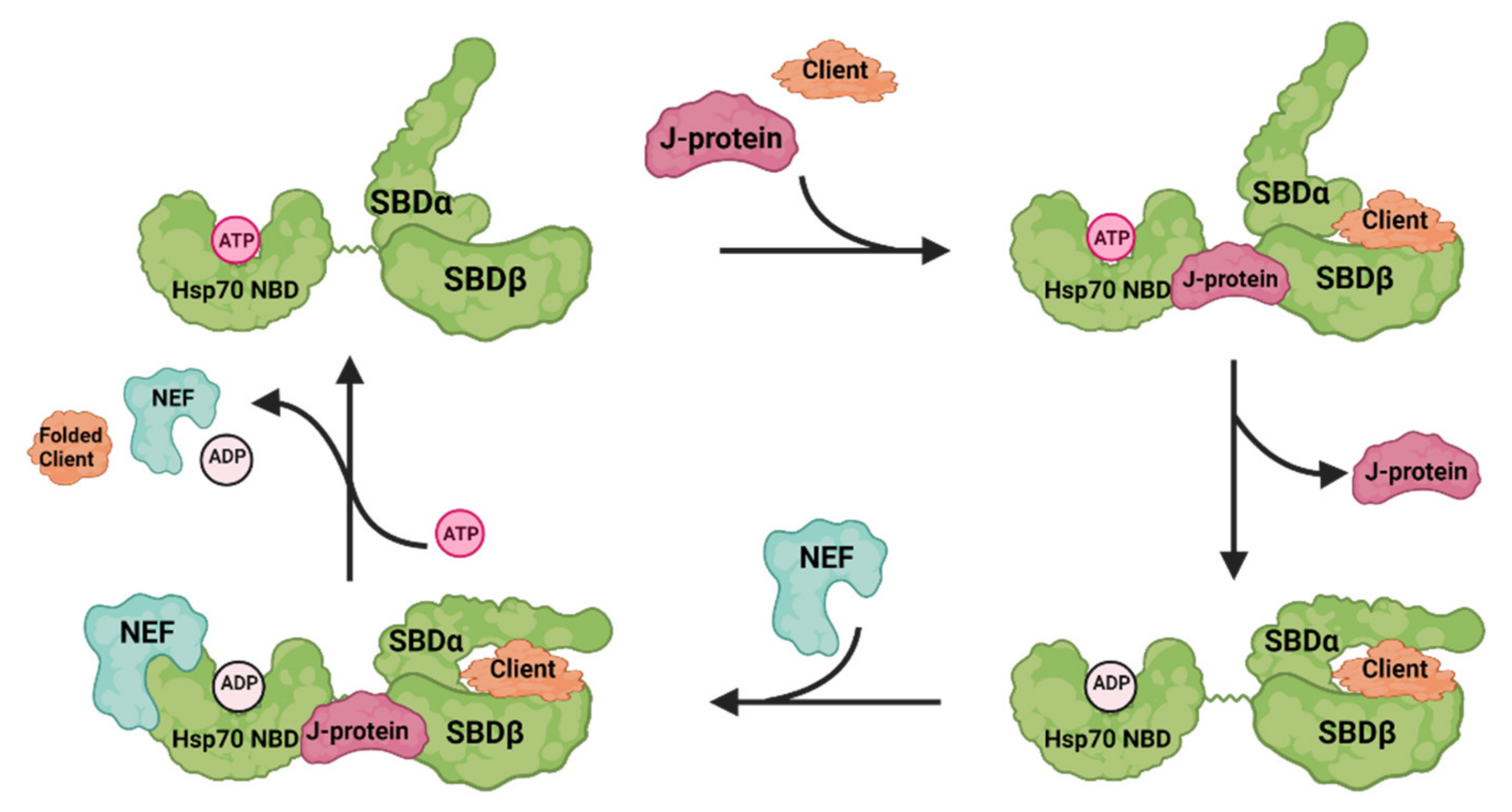This is a detailed diagram seemingly taken from a biology textbook, illustrating the intricate cycle and interactions of various protein structures, meticulously labeled and color-coded for clarity. At the center top of the diagram, prominently highlighted in pink, is the J-protein, a key player in the sequence, alongside an orange-shaded client protein. The diagram is a flow chart, marked by black arrows that guide the viewer through different stages and interactions involving the proteins.

The J-protein and client complex first interact with HSP70, another protein, which is depicted in green, along with ATP, colored in pink. This complex also includes SBD-alpha and SBD-beta segments. Moving along the flow chart, the diagram shows a transition as ATP converts to ADP, represented in white, and involves additional structures like NEF, illustrated in blue.

The flow chart further demonstrates how these molecules interchange components, such as exchanging ATP for ADP and aligning with NEF. Arrows guide through multiple transitions, showing connections among J-protein, HSP70, and various client states like ‘folded client,’ highlighting their dynamic interactions. 

Each element, such as the SBD-alpha (green), SBD-beta (green), and the various states of the client protein (orange), is distinctly labeled and color-coded to facilitate understanding. The shapes depicted are irregular and somewhat jagged, emphasizing the natural complexity and organic form of these molecular structures. The ultimate goal of the diagram is to visually convey the flow and interaction paths of proteins, ensuring that the fundamental processes within cellular biology are clear and comprehensible.